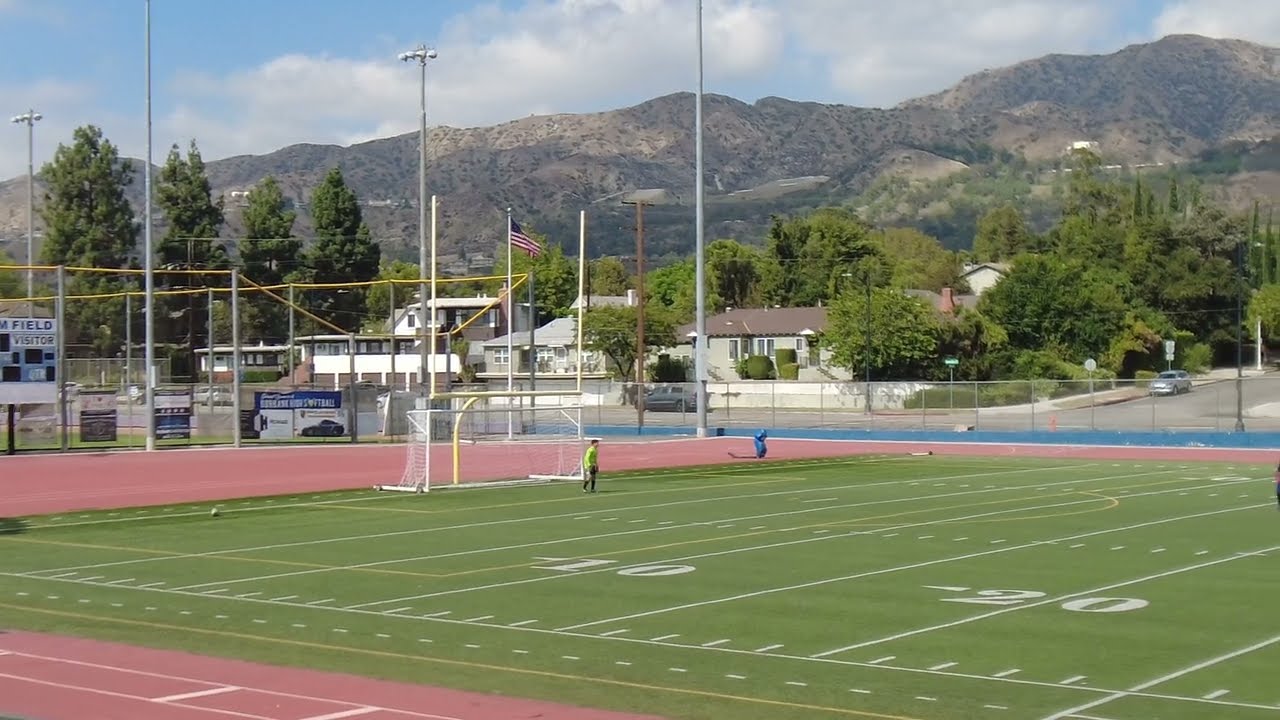The image depicts a large, green football field bordered by white lines and numbers, specifically -10 and -20. Surrounding the field is a red (or pinkish) track, with a yellow field goal post and a white soccer net below it at one end. A man in a bright greenish-yellow jacket and gray pants is walking on the grass, while another person in a blue shirt is seen near the middle gate. In the background, a neighborhood of houses and apartment buildings nestles among a variety of green trees, including both regular-sized and tall, slender pine trees. Beyond the neighborhood rise tall brown mountains with a blue sky and white and gray clouds above, completing the scenic backdrop. A metal fence around the field, traffic signs, a sidewalk, and a car on a side street further detail the setting.